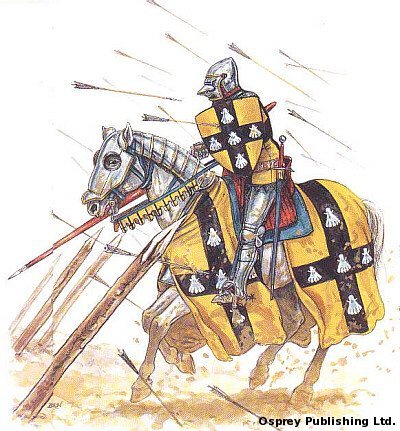This colored pencil drawing vividly depicts a Middle Ages knight in silver-gray chain mail and plate armor aboard his imposing destrier, a warhorse. Both the knight and horse face left against a pristine white background, poised as if ready for battle. The knight, with a guard-plated helmet, brandishes a long orange lance in his right arm while a yellow shield with a brown cross and white emblems rests on his left arm. Mirroring this design, a yellow blanket adorned with brown crosses and white symbols drapes over the horse's back, covering its armored neck and chest. The horse stands in a charging stance with stirred dust beneath its hooves, its right leg straight and its left leg raised. Surrounding them are sharp wooden spears protruding from the yellow ground and a flurry of arrows flying overhead and embedded in the earth. A subtle watermark in the bottom right corner identifies the illustration's origin as Osprey Publishing, LTD, adding to the sense of historical authenticity.